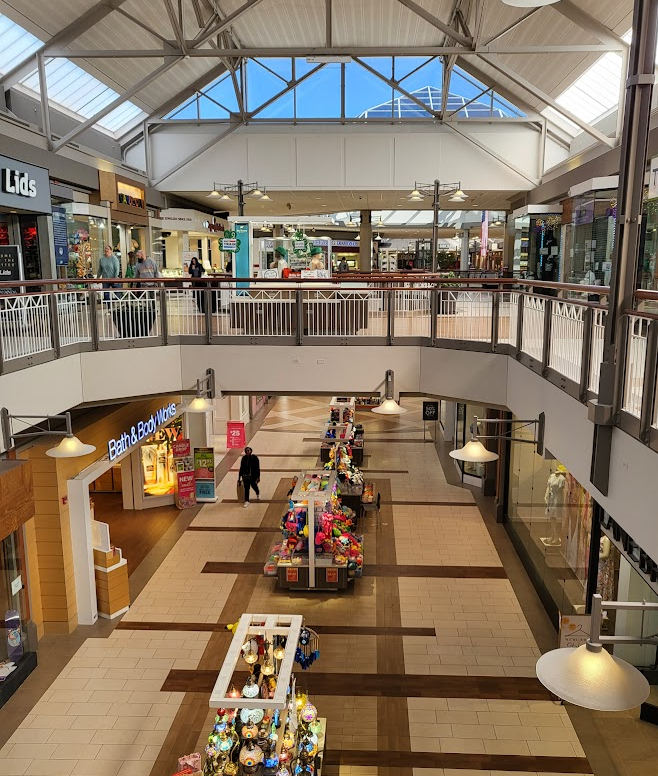This image captures a bustling, well-lit shopping mall viewed from the second floor. The mall features two levels, with the ground floor characterized by a mixture of light cream-colored bricks and brown highlights, including a wooden-looking section running down the middle. In this central aisle, various small stands display different items for sale. A Bath and Body Works store is prominently located on the lower left side, near which a person is walking. The floor itself is tiled, combining light colors with dark brown and light brown patterns.

Further adding to the ambiance, lamps are suspended from the walls of the second floor, illuminating the ground level. Moving up, the upper floor has more foot traffic, with notable shops such as Lids on the left. The second floor is detailed with a brown railing over white vertical bars, with seating areas visible just beyond it. 

At the top of the image, the roof, partially metal with skylights, opens up to reveal glimpses of the blue sky and sunshine streaming in from the upper right. Above the shops, windows provide views of another building in the distance, possibly part of the same complex or a separately adjacent structure. The ceiling design also features large pieces supported by beams, adding architectural interest. Overall, this lively scene is reminiscent of a typical, vibrant mall from an earlier time, where most stores remain occupied and busy.